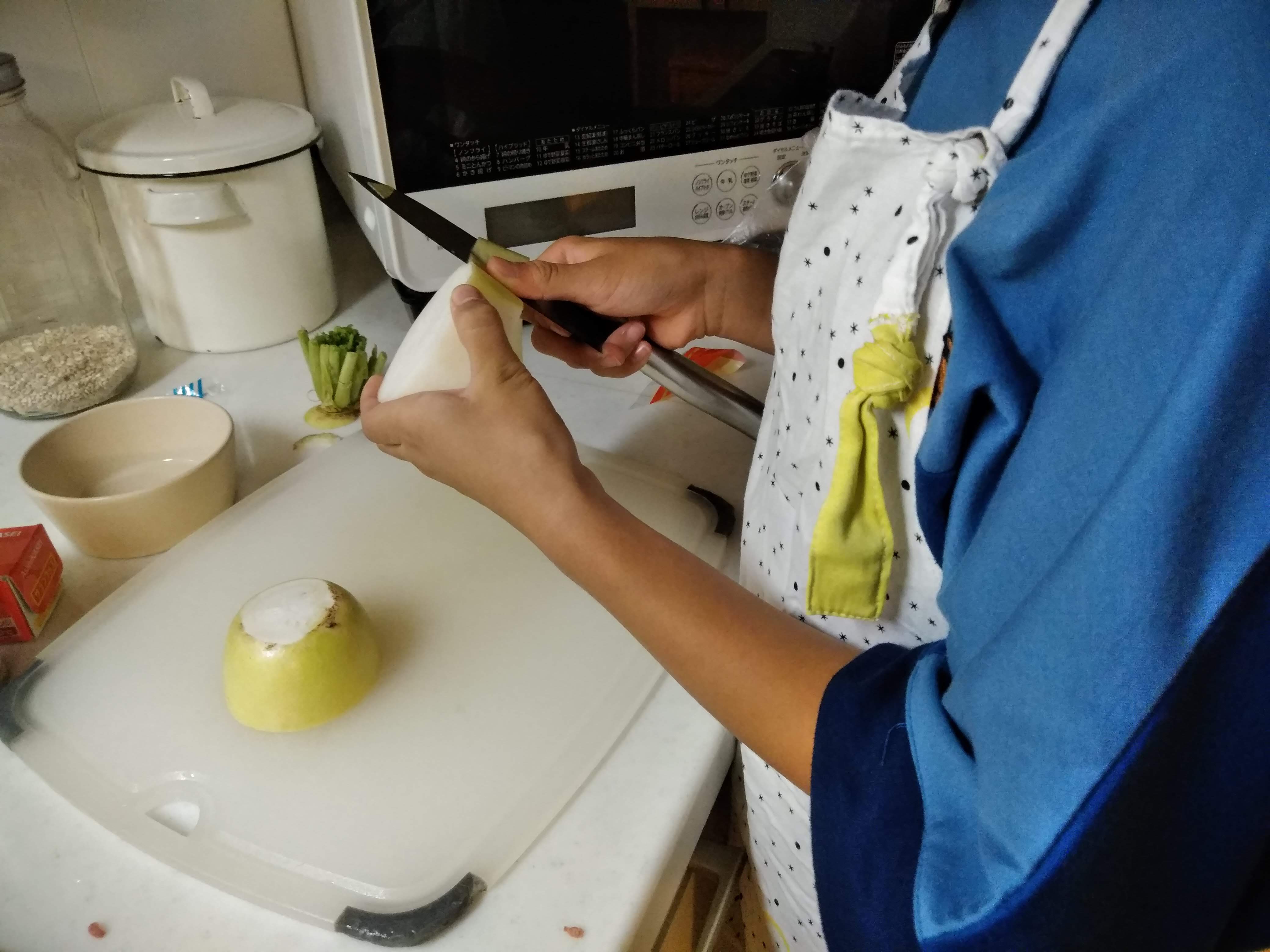In a cozy kitchen setting, a person is intently focused on preparing vegetables at a cutting board. She is meticulously peeling a white, tuberous vegetable with a paring knife, which bears a resemblance to a potato but isn’t one, as evidenced by its carrot-like green top set aside with the unpeeled slice nearby. She is almost finished with the piece in her hand. Clad in a charming apron adorned with blue, gray, and possibly off-gold polka dots, she pairs it with a blue satiny shirt featuring navy blue sleeves that reach her elbows. To the right of her workspace, a microwave and several canisters create a homey backdrop, supplemented by a bowl placed just beyond the cutting board, hinting at more kitchen tasks ahead.